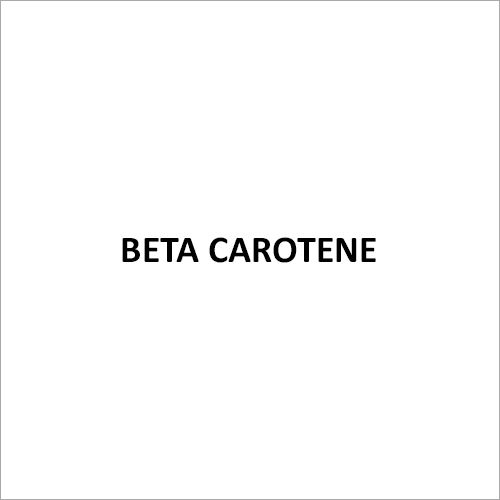The image is a simple, white square with a very thin light gray border. At the center, written in clear, black, uppercase letters are the words "BETA CAROTENE" (spelled out as B-E-T-A space C-A-R-O-T-E-N-E). The text, located centrally within the square, is relatively small, estimated to be less than one-tenth of the square's total height. The surrounding white space is ample and balanced, with roughly an inch of space to the left and right, and about two to five inches above and below the text. The design is minimalistic, featuring no additional images, colors, or background elements, emphasizing the simplicity and clarity of the typography.